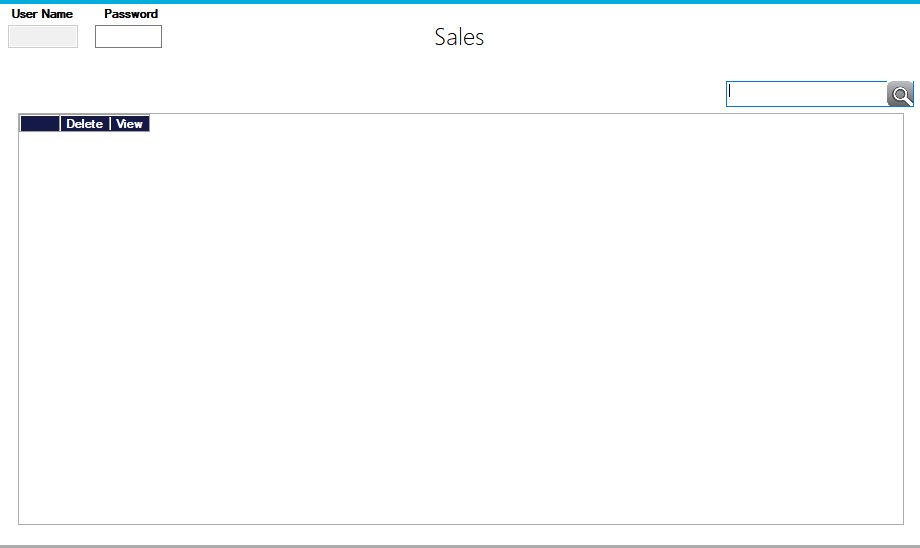This image is a cropped screenshot of a sales program interface. At the very top, the word "Sales" is prominently displayed in black font, serving as the title of the page. In the upper left corner, there is a section for user authentication. It includes the labels "Username" and "Password," both in bold black font with corresponding empty input boxes below them.

Adjacent to these fields on the right side is a search box, although the magnifying glass icon typically found within or next to it is partially cropped out, suggesting the image has been truncated on the right edge. The central area of the screenshot is largely blank, signifying an unpopulated form on a white background.

In the upper-left corner, a row of three blue buttons is visible. The first button is simple and unlabelled, while the second button is labeled "Delete," and the third one is labeled "View." Additionally, subtle guidelines structure the interface. A blue horizontal line runs across the top, and a gray horizontal line runs across the bottom, framing the content area.

The overall composition indicates a user-friendly, minimalistic design focused on essential functions like user login and search capabilities.